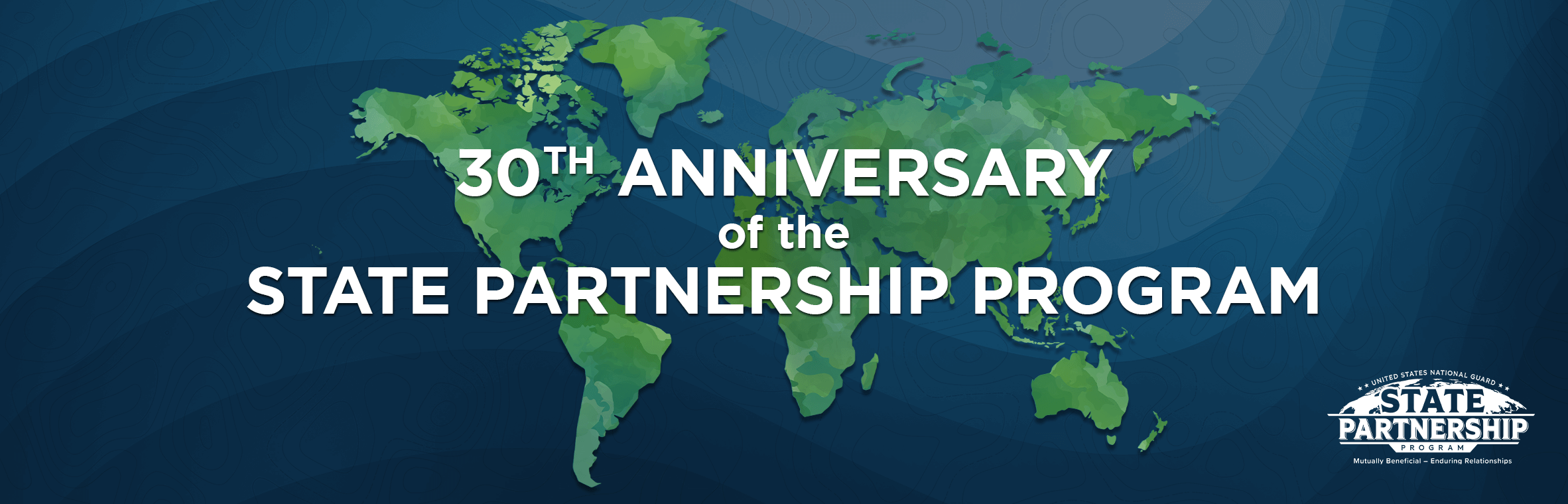The image is a computer-generated promotional poster celebrating the 30th anniversary of the State Partnership Program. The background is a dark blue, representing the Earth's oceans, with a green world map showing the continents. At the center of the image, bold white text reads "30th Anniversary of the State Partnership Program," with the 'TH' in "30TH" presented in a superscripted sans-serif font. In the lower right corner, there is a logo with the words "State Partnership," where "State" appears in dark blue and "Partnership" is in white against the dark blue background. The overall design emphasizes a global celebration, signifying the program's widespread impact across all continents.